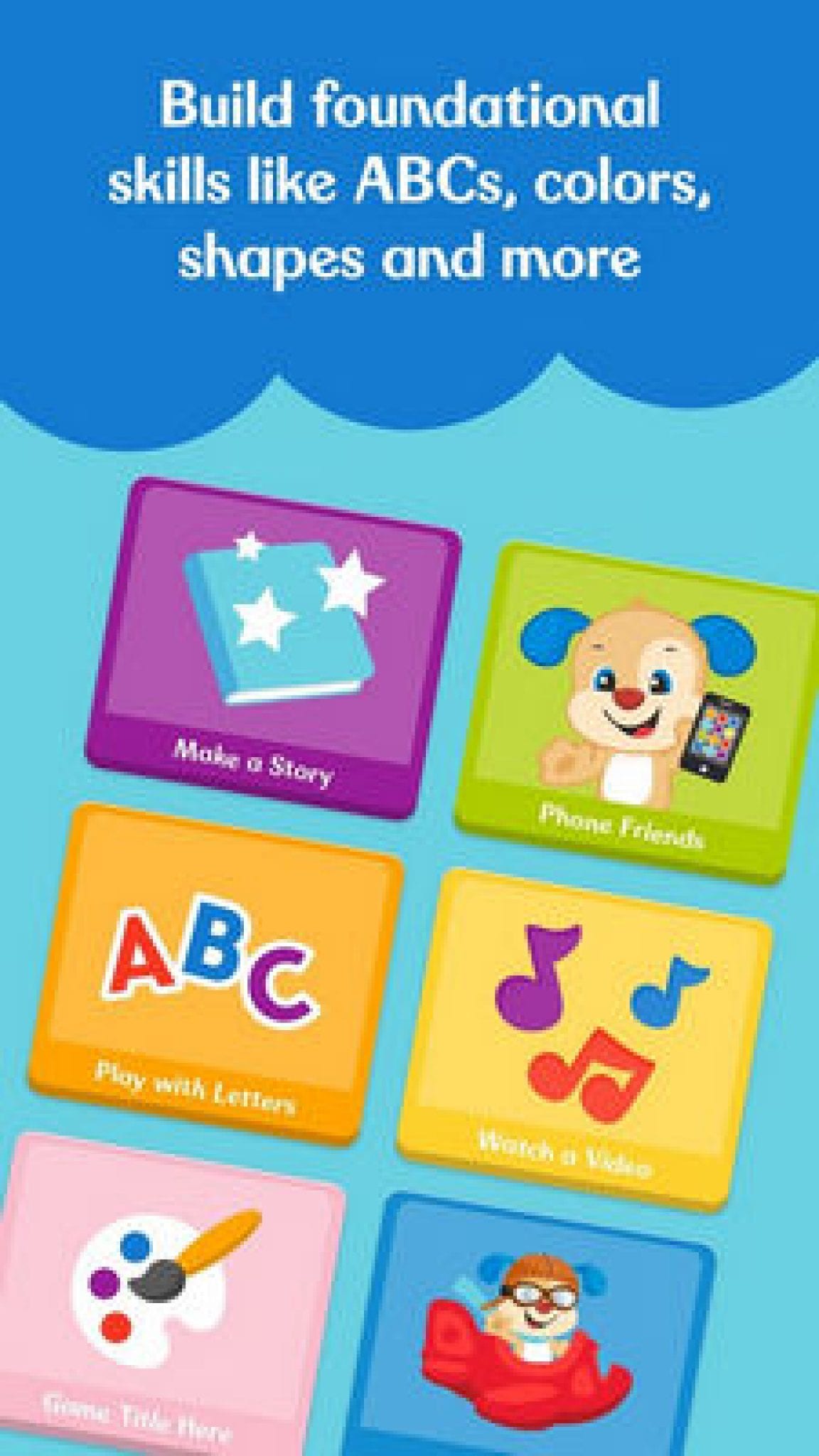An educational graphic displays multiple elements designed to promote foundational learning skills for children. The background features a gradient of light blue with bumpy textures at the bottom, transitioning to a pattern of squares. Prominently, a book with the phrase "Make a Story" in purple text is centered, accompanied by three white stars above it.

In the bottom left corner, a cartoon dog with blue ears and black edges is shown holding up a phone, with "Phone Friends" written in the center of the device. Surrounding the dog are various text elements in vibrant colors: orange, red, blue, and purple proclaim different learning activities. The caption highlights basic skills like ABCs, colors, and shapes.

On the right side of the image, a colorful paint palette and brush are displayed against a pink backdrop, promoting creative activities. Further to the right, a plane with another dog character in blue is positioned at the center, suggesting an adventurous aspect of learning. Additional text says "Watch Video," indicating multimedia content to support interactive learning.